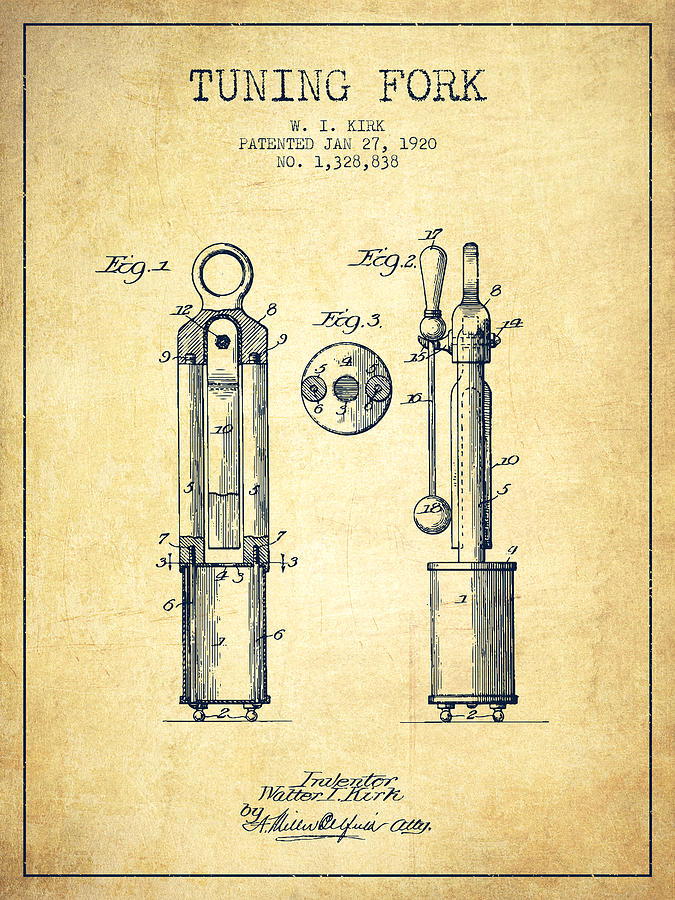This detailed image is an antiqued illustration on tan-colored parchment paper, likely part of a patent application, depicting a tuning fork device patented by W.I. Kirk on January 27, 1920, with patent number 1,328,838. The drawing, rendered in black ink, features two labeled figures—Figure 1 and Figure 2—possibly showing different views or mechanical aspects of the tuning fork. At the top, the text "Tuning Fork" is prominently displayed. The device includes components such as a lever and a heavy ball, which might be used to produce specific sounds for tuning purposes. Despite its intricate design, there are no indications of motion, leaving the exact functionality somewhat unclear. The document also mentions "Inventor Walter Kurth" and lists an attorney submission. The overall style and aged appearance of the paper lend a historical, scientific aesthetic to the illustration.